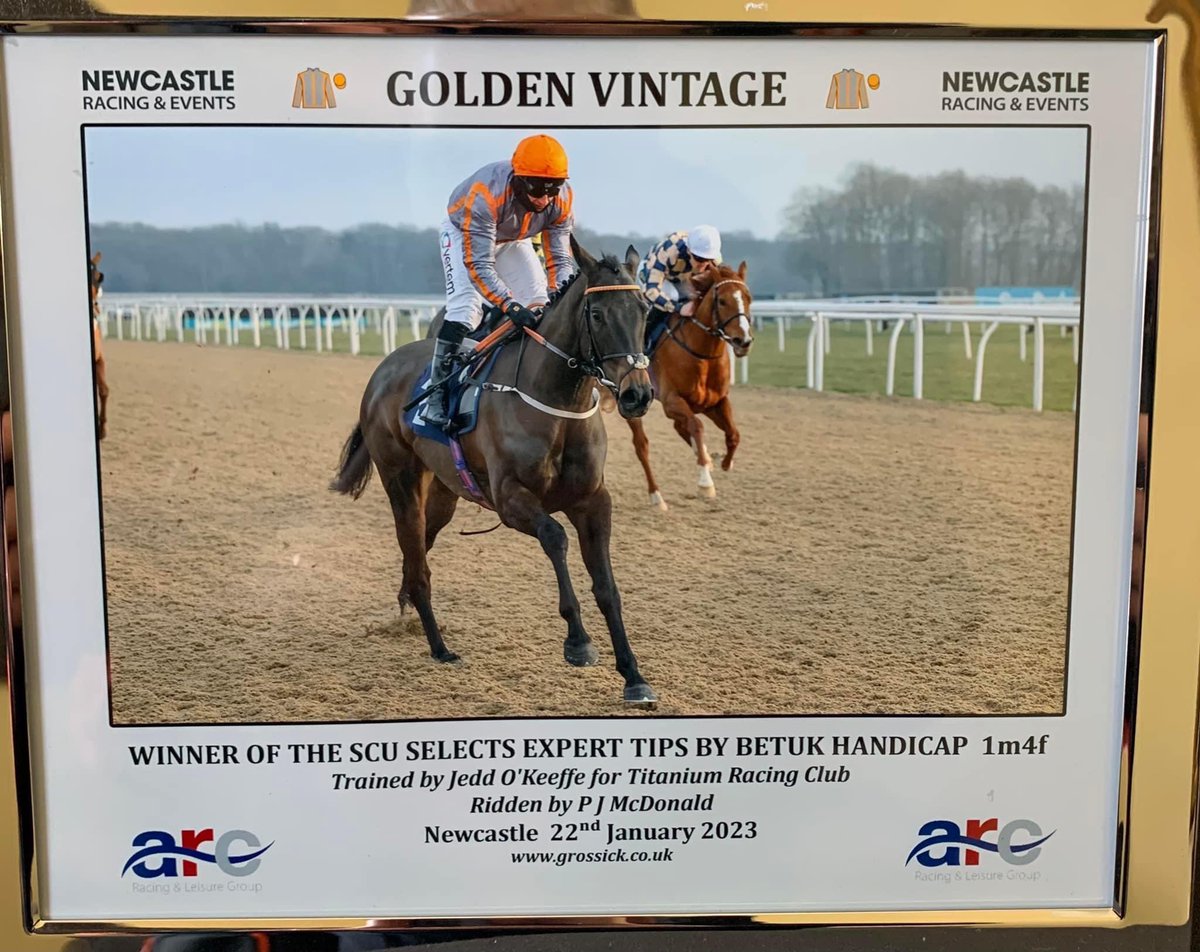The image showcases a polished brass frame, narrow at the top and bottom but wide on the sides, housing a color photograph bordered by a white edge. At the top of the border, the text reads "Newcastle Racing and Events - Golden Vintage," accompanied by a small drawing of a jockey's helmet and top. The central photograph captures a lively horse race on a dirt track, with a white perimeter fence, verdant fields, and rows of trees in the background. 

In the forefront, a jockey in an orange helmet, gray jersey with orange stripes, white pants, and black riding boots stands in the stirrups over a dark brown horse, likely leading the race. Beside him, another jockey, clad in a white helmet and a salmon-and-dark harlequin checked jersey, rides a chestnut brown horse. The bottom of the photograph details the event: "Winner of the SCU Selects Expert Tips by BetUK Handicap. One mile, four furlongs. Trained by Jed O’Keefe for Titanium Racing Club, ridden by PJ McDonald. Newcastle, 22nd January 2023." The internet address www.grosick.co.uk is also displayed, alongside the ARC symbol in the lower corners.